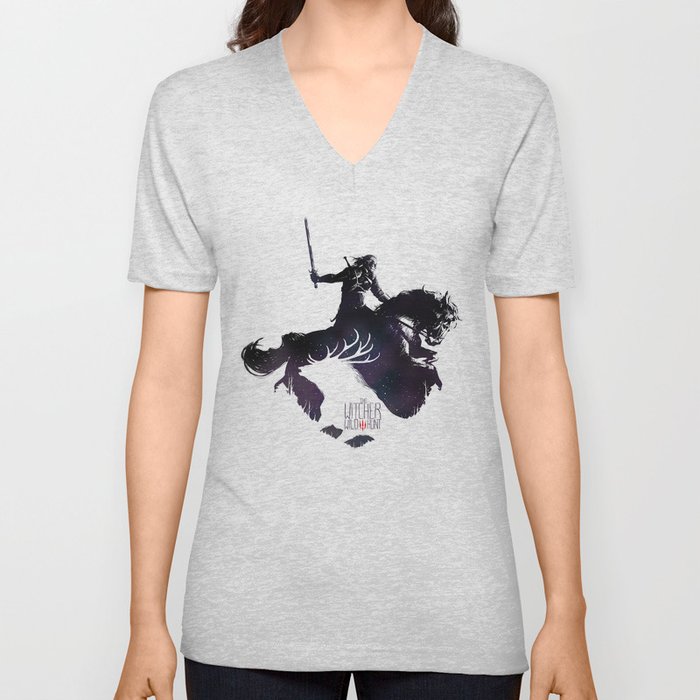This image showcases a young Caucasian woman with long dark brown hair, modeling a light heather gray, deep v-neck, short-sleeve t-shirt against a gray background. Her face is not visible, as the view is from her neck down to the top of her thighs. She is wearing dark blue jeans with the t-shirt. The t-shirt features an intricate black design depicting a figure with long hair, possibly a warrior or a knight. The figure is mounted on a mythical, horse-like creature with fluid, blurred legs, a flowing mane, and a tail. The warrior is holding a drawn sword in their right hand while their left hand grips the creature’s mane or reins. Superimposed over this scene is a silhouette of a large-antlered creature, similar to a moose or deer. Below the design, in small text, it reads, "The Witcher Wild Hunt."